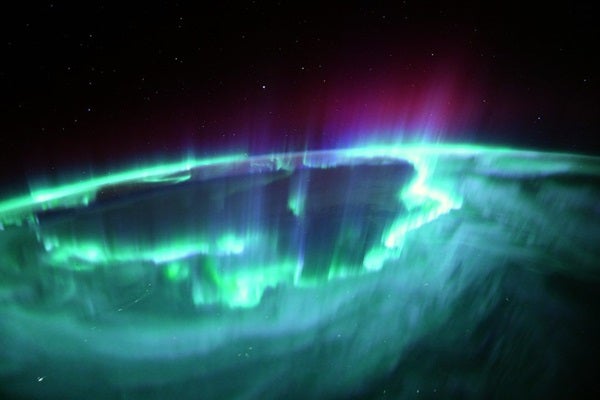The image captures a stunning astronomical phenomenon featuring an aurora, likely the Northern Lights, displayed against a stark black night sky. Dominating the scene is an uneven, wobbly ring of green light, glowing vibrantly over a blue planet, though the exact celestial body remains unspecified. The green light varies in intensity, with sections of neon green juxtaposed against darker, gassy green areas, forming a circular shape with a dark, irregular hole at its center. Enhancing the visual spectacle are streaks of blue and purple light that shoot vertically, adding to the ethereal beauty of the scene. The top of the image features the blank expanse of outer space, dotted with tiny white speckles representing distant stars. This high-contrast, color-enhanced photograph showcases celestial photography at its finest, offering a mesmerizing view of space and light.